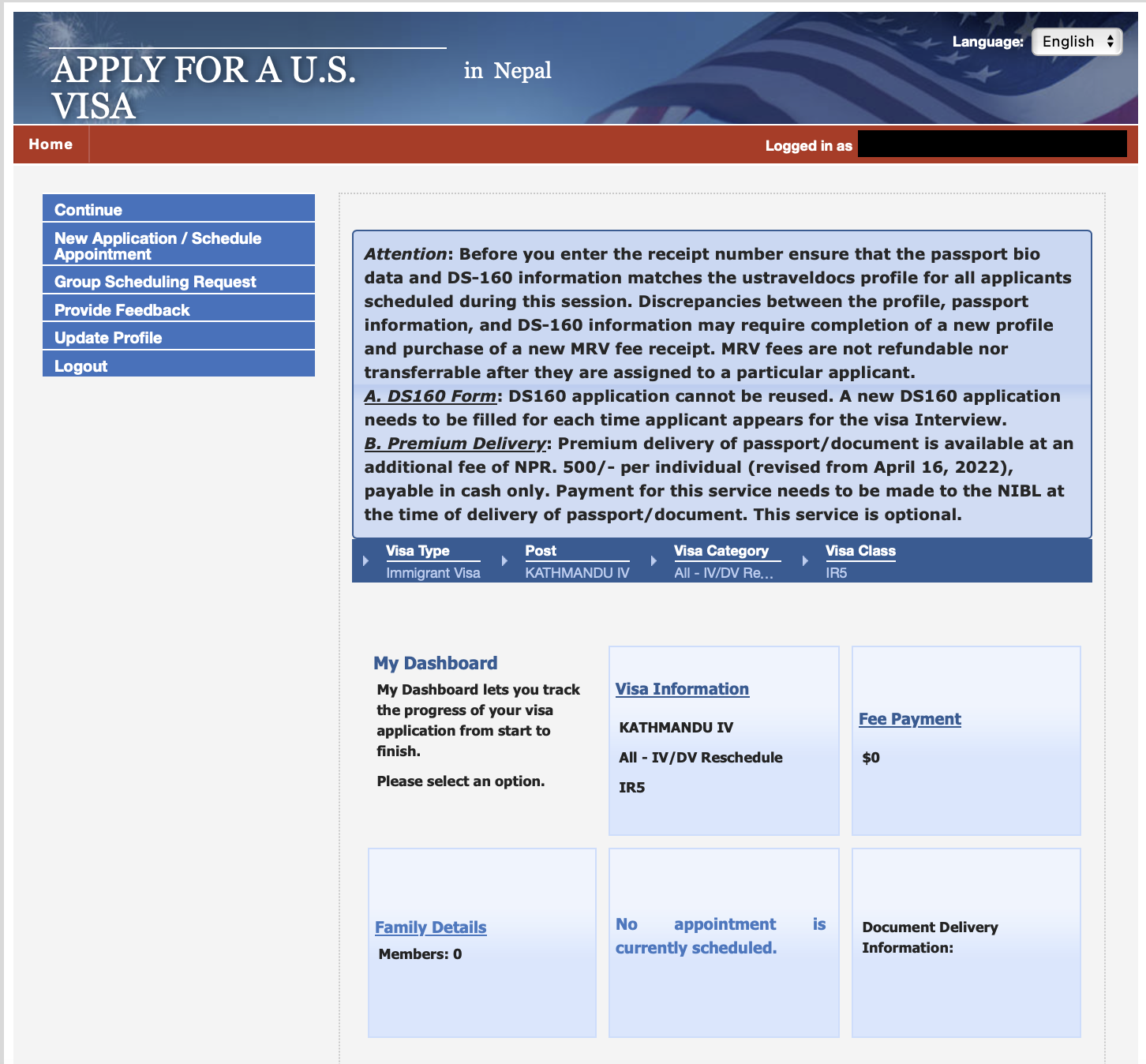This is a screenshot from a webpage designed for applying for U.S. visas in Nepal. The header features a blue bar with a small U.S. flag icon in the top right corner. In this bar, white text reads, "Apply for a U.S. visa in Nepal," and just below it, the language is indicated as "English." 

A prominent red bar spans the screen below the blue header. On the left side of this red bar, it says "Home," while on the right, it indicates "Logged in as," followed by a blurred-out username to maintain privacy.

The main content area of the webpage has a clean white background. To the left, there is a vertical menu composed of blue rectangles featuring various options: "Continue," "New Application/Schedule Appointment," "Group Scheduling Request," "Provide Feedback," "Update Profile," and "Log Out."

In the central portion of the screen, a large blue rectangle commands attention with essential information. It instructs users to ensure that the passport bio-data and DS-160 information match the U.S. Travel Docs profile for all applicants scheduled during the session. It warns that discrepancies among the profile, passport information, and DS-160 may necessitate creating a new profile and purchasing a new MRV fee receipt. It also notes that MRV fees are non-refundable and non-transferable once assigned to an applicant.

Additionally, the notice highlights two key points:
1. **DS-160 Form** - The DS-160 application form cannot be reused, and a new form must be submitted for each visa interview.
2. **Premium Delivery** - This option is available for an extra fee of NPR 500 per individual, updated as of April 16, 2022. Payment is cash-only and must be made to NIVL at the time of passport delivery. This service is optional.

Below the notice are several options for navigating the system: "My Dashboard," "Visa Information," "Fee Payment," "Family Details," and "No appointment is currently scheduled," followed by "Document Delivery Information."